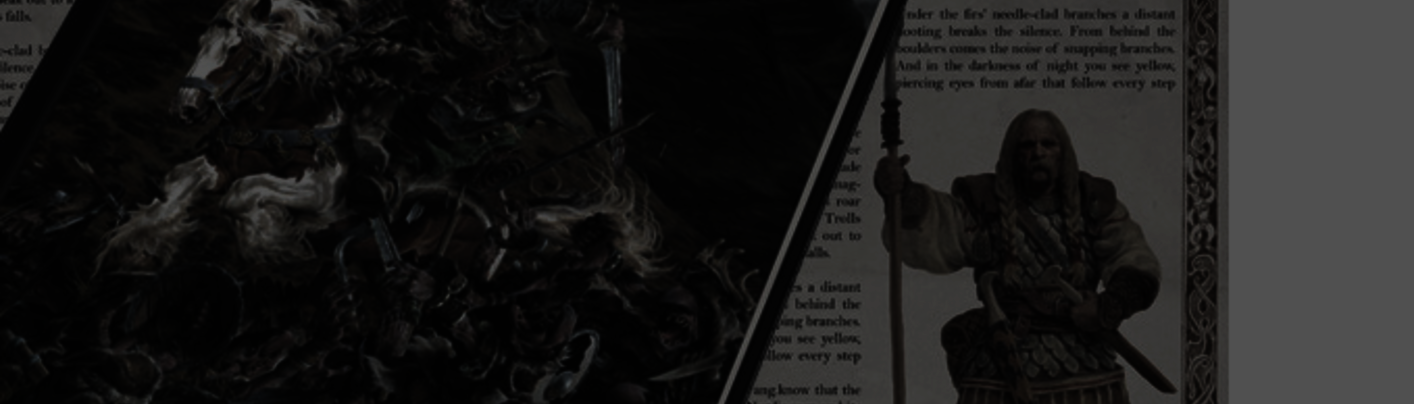This horizontal rectangular image, taken in very low light, features a large, dark-colored book with a predominantly black cover. The title "True Dwang Chronicles" is printed in white text, accompanied by the name "Riot Minds" on the cover. The design on the cover depicts a warrior riding a horse. Positioned centrally in the image, the book rests on what appears to be a gray surface. Behind the book, an open page or poster is visible, showcasing an illustration of a man who resembles an old Viking warrior, wielding a sword and a spear. The poster has designed borders on all sides and is filled with text that is not legible due to the low light conditions. The overall color scheme of the image is black and white, with interesting and colorful fonts that enhance the aesthetic despite the darkness.